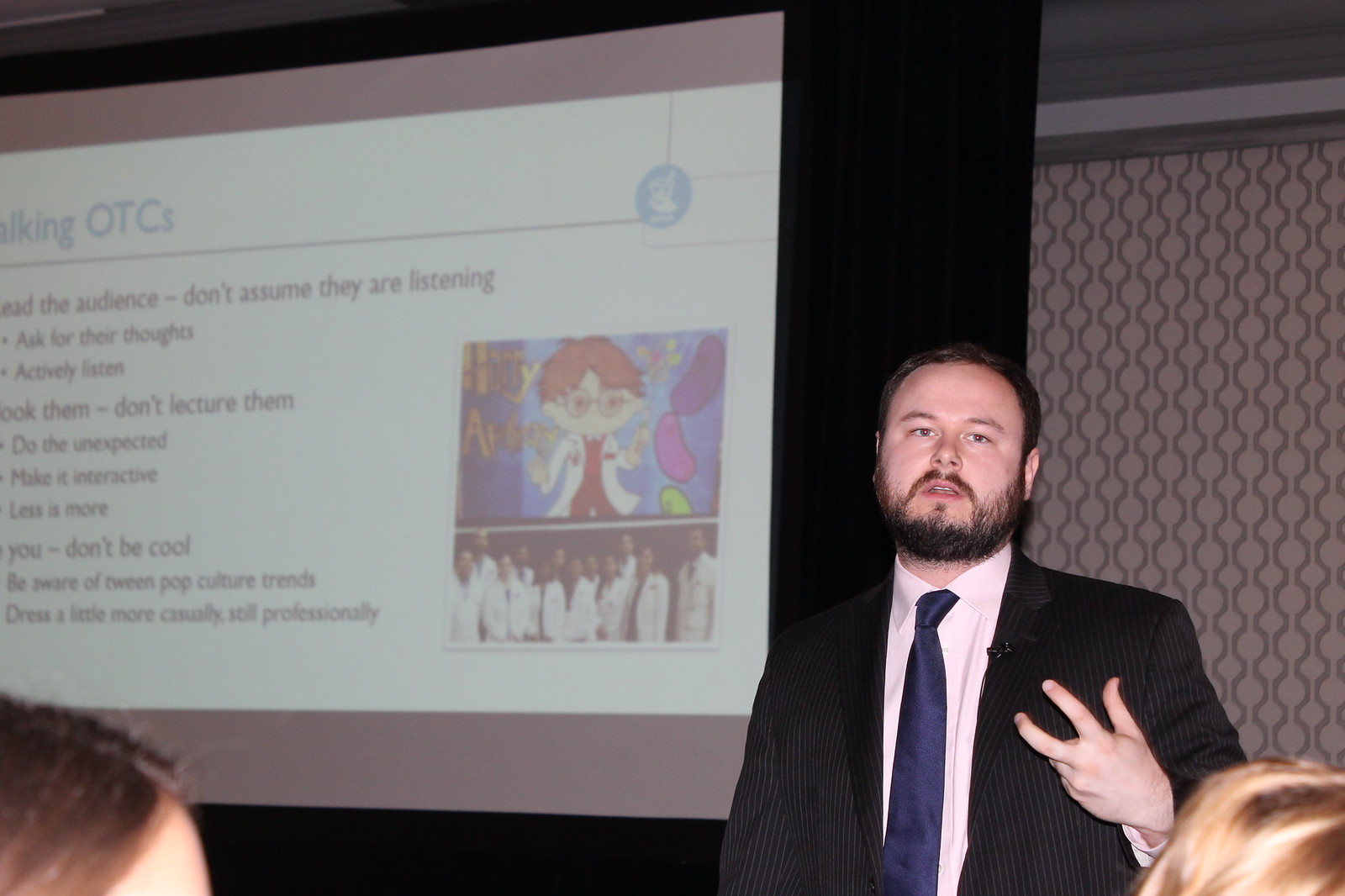In this semi-dark, indoor setting, likely a hotel conference hall, a man wearing a black suit jacket, white button-up shirt, and blue tie stands at the bottom right corner of the image, delivering a presentation. He gestures with his left hand and has a light beard and short hair, with a microphone pinned to his lapel. Two audience members are partially visible in the lower corners of the image—the top of a blonde head on the right and the top of a brunette head on the left. The background features a patterned wallpaper, and to the left, a projector screen displays a mix of faded and unreadable text along with two discernible images: a cartoon character with glasses and a lab coat, and a group of people in white lab coats, suggesting a scientific or medical theme. The overall ambiance is dark enough to allow the projection to be visible but still provides enough light to see the room's details.